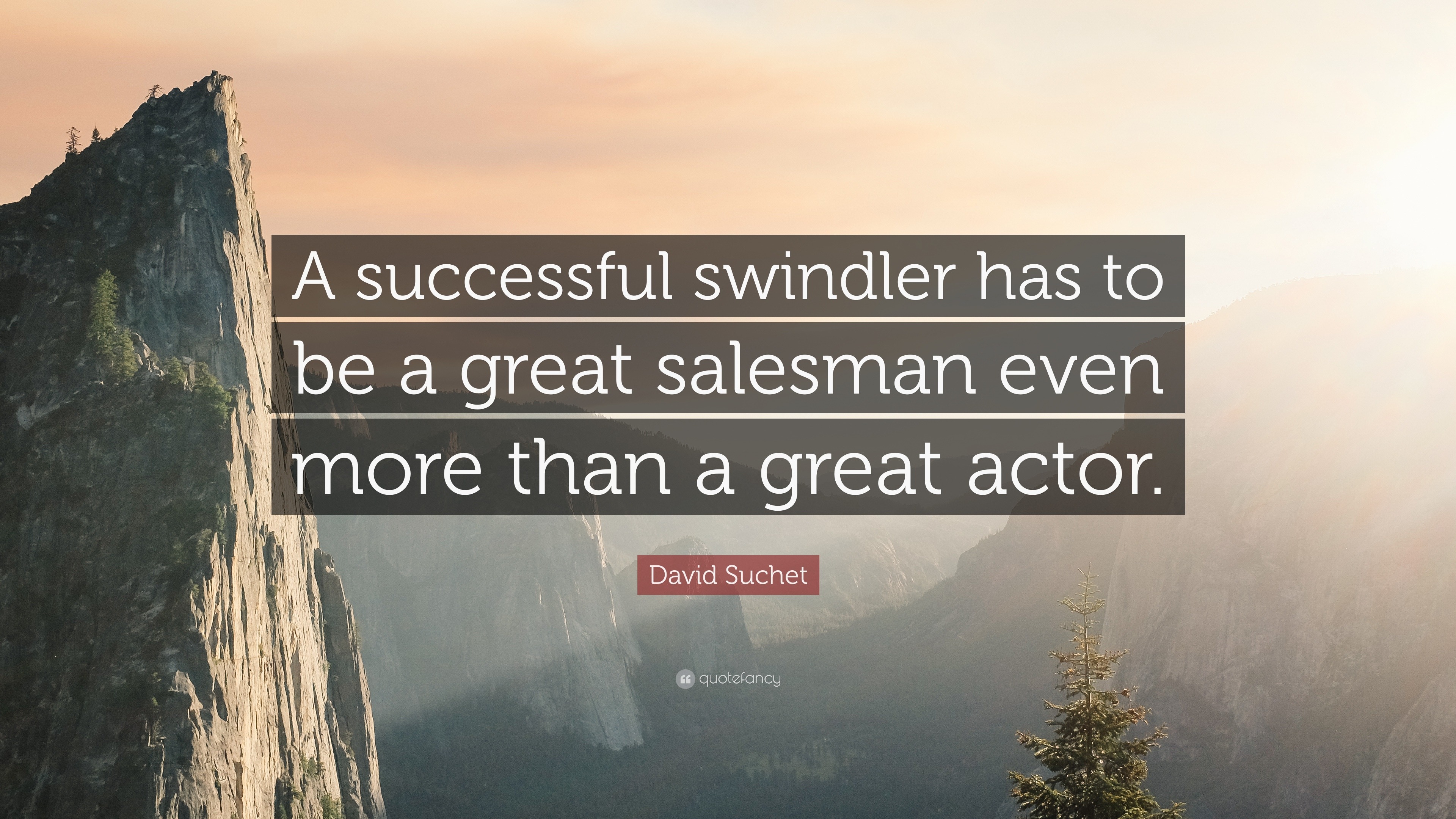The image is a stunning, high-resolution photograph of a mountainous landscape, likely inspired by the Alps. Jagged, rocky peaks dominate the scene, with the tallest peak on the left casting a prominent shadow. To the right, the sun is setting behind another mountain, casting a brilliant golden hue across the sky which blends with shades of orange, yellow, and gray due to the reflected light from the clouds. 

Midway through the image, three semi-transparent black bands overlay the mountains, each progressively wider and featuring white text. The inspirational quote reads, "A successful swindler has to be a great salesman even more than a great actor," attributed to David Suchet, who is noted for his portrayal of Hercule Poirot. Below the quote, against a translucent red rectangle, lies the attribution "David Suchet." At the very bottom of the image in smaller white text is the label "quote fancy," indicating the source of the quote design. 

Despite the textual overlay, the background remains a captivating, serene view of rugged peaks, flowing valleys, and sparsely distributed trees, all illuminated by the warm, celestial light of the setting sun – a composition that would indeed make for an inspiring screensaver or poster.